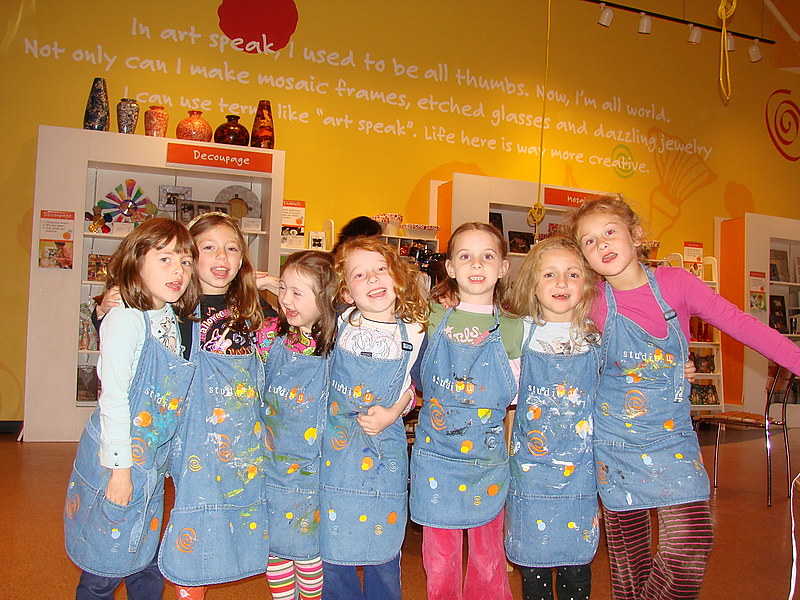This indoor photograph captures a lively group of 7 young girls posing happily for the camera. They stand closely with broad smiles, each wearing a blue apron that seems designed to protect their clothes, suggesting they are in an art studio environment. The background features a vibrant yellow wall adorned with text in white that reads, "In art speak, I used to be all thumbs, now I am all world. Not only can I make mosaic frames, etched glass, and dazzling jewelry, I can use terms like art speak. Life here is way more creative." The wall also displays various drawings, adding to the creative atmosphere. Adjacent to the wall, shelves are filled with decorative items, emphasizing the artistic setting. A solitary chair is visible on the brown-colored floor on the right side of the image. Overall, the scene vibrantly captures the joyful and creative spirit of the young artists in an engaging art studio.